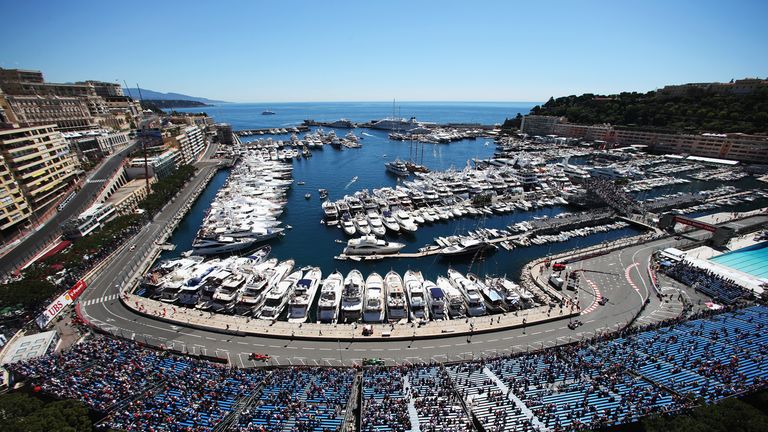This above-view photograph captures a vibrant, tropical marina surrounded by a Grand Prix-style racetrack lined with curbs and bends, nestled within a cityscape. Central to the image, a multitude of white yachts and cabin cruisers are neatly aligned on the serene, blue waters. A significant grandstand, filled with dots resembling people, occupies the lower portion of the image, overlooking the racetrack and marina. The track loops around the marina, and tiny racecars can be seen zipping by. To the right, lush green trees and a separating wall border the marina. Above this bustling scene, a clear, cloudless blue sky stretches across the horizon, enhancing the tropical, vacation-like atmosphere.